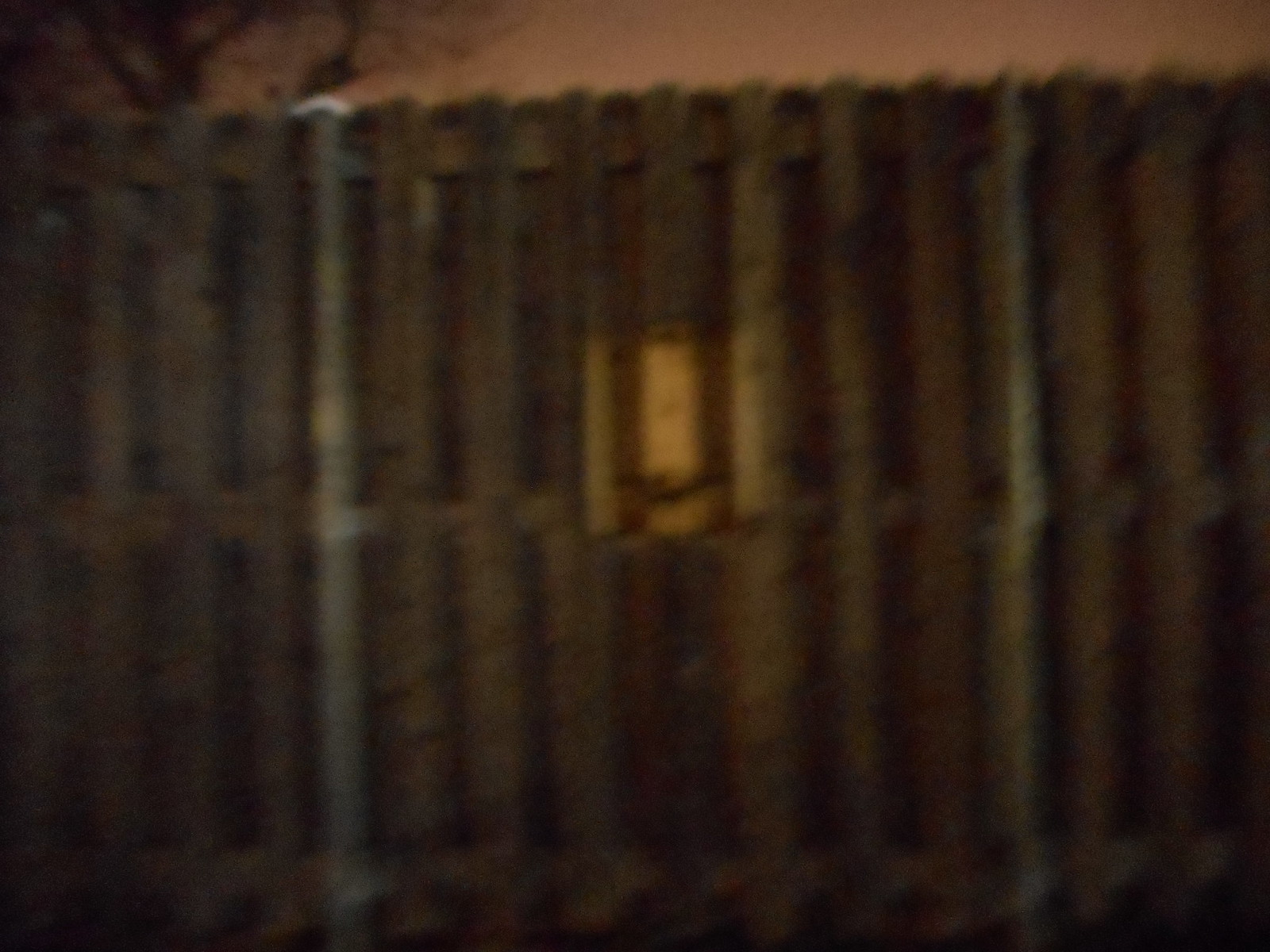The image is a zoomed-in, blurry close-up of a tall wooden fence. The fence consists of numerous vertical wooden slats, about 12 in total, with three horizontal beams reinforcing them—one at the top, one in the middle, and one at the bottom. Additionally, there are two silver-like bars spaced evenly, one-third from the left and one-third from the right. The photo appears to have been taken at night, making the image rather dark, but the details are still distinguishable. Near the center of the fence is a small, barely identifiable square object with a yellowish hue, possibly a sign. Above the fence, in the upper part of the image, there is a visible portion of a tree trunk and branches that are bare, suggesting a winter season. The upper part of the image also has a pinkish-brown or beige coloration, which might be the outline of a nearby roof or structure. The image gives an impression of being taken in an urban setting, possibly just above a subway entrance in a city like New York.